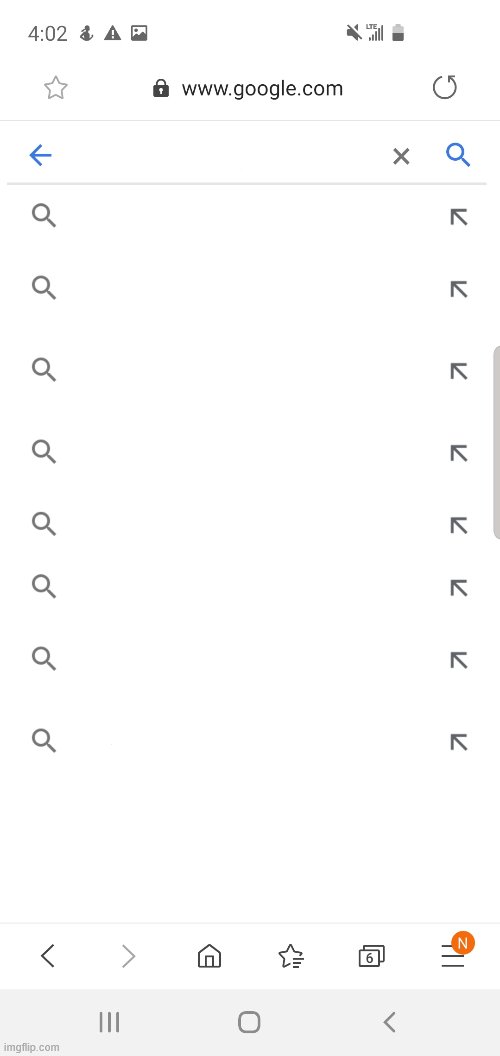This detailed caption avoids unnecessary repetition and provides clear descriptions of the icons and elements present in the smartphone screenshot.

"Screenshot of a smartphone displaying the website www.google.com. At the top of the screen is a timestamp reading '4:02' accompanied by three icons. The first icon is unidentified, the second resembles a warning symbol, and the third appears to be a picture icon. To the far right are a volume icon indicating it is off, an LTE signal indicator, and a battery icon showing about half charge.

Below this bar, to the left, is a star icon next to the URL 'www.google.com' with a lock symbol to the left, indicating a secure connection. To the right of the URL is a refresh arrow. Directly beneath is a navigation toolbar consisting of a left-facing blue arrow, a close-out 'X', and a search bar.

The search bar precedes eight search icons, followed by vertical arrows, displayed from bottom right to top left. At the bottom of the screen, there is a navigation bar featuring a left-facing arrow, a right-facing arrow, a home icon, a star icon, and a pages icon. At the far right end of this bar is a hamburger menu icon with an orange circle containing the letter 'N'. Lastly, below this bar are a home button, a close-page button, and a left-facing arrow."